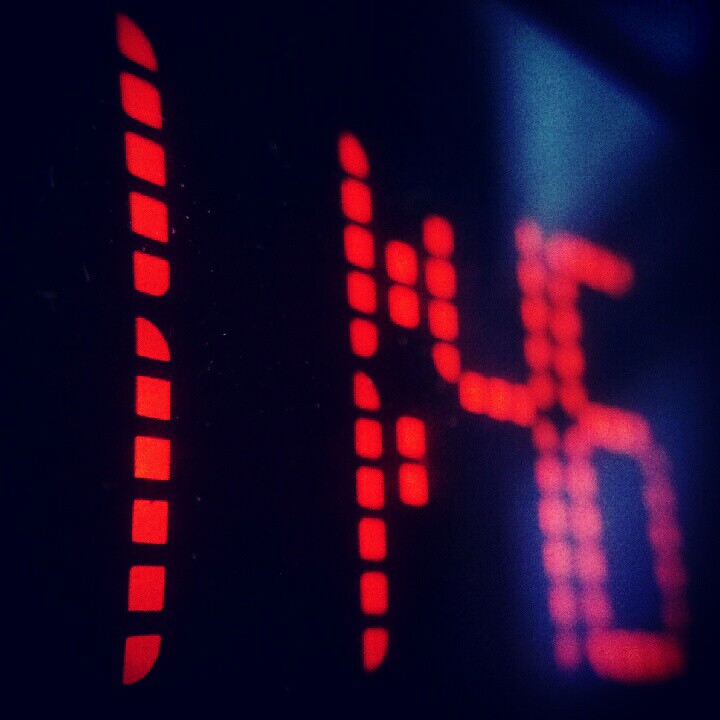The image shows a close-up view of an electronic digital clock display. The photograph is so magnified that it becomes challenging to identify the device accurately. The background is pitch black, creating a stark contrast that highlights the red digital numbers. The clock display is slightly diagonal, tilting more towards the bottom left, with more of the black background visible on the right side. The digital numbers appear as if created by red dots or red segments forming squares. The visible time reads "11:46," but there is no indication of whether this is in the morning or evening (a.m. or p.m.).